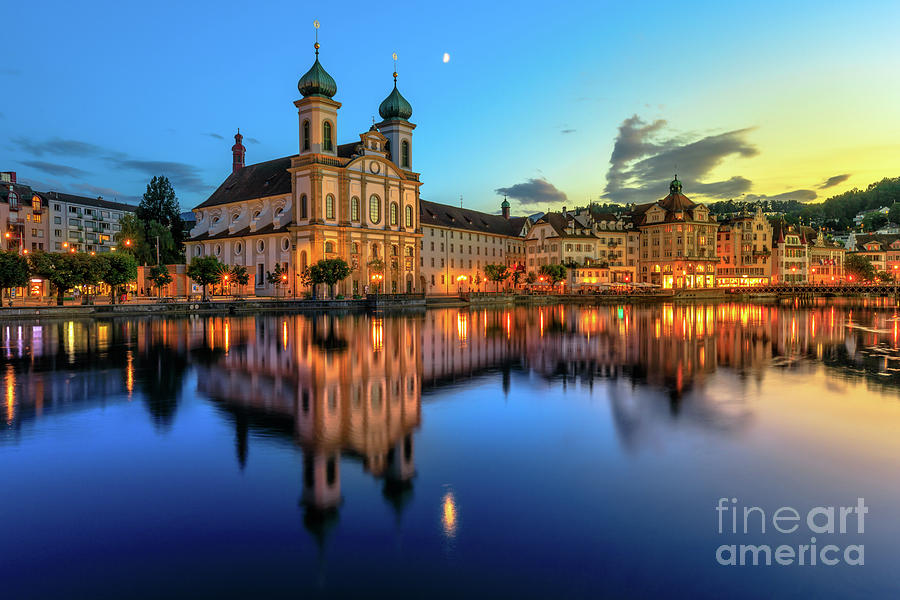The photograph captures an evening scene with a serene body of water in the foreground, possibly a lake, reflecting its surroundings. The water, dark blue in the center and lighter to the right, mirrors an array of cream-colored, European-style buildings, some adorned with green onion domes that resemble Hershey's Kisses, likely indicating churches. Prominently, a palatial building with twin steeples stands out, its architectural details clearly visible. Along the shoreline, trees and streetlights mix with the buildings, their lights twinkling and contributing to the reflections on the water's surface. The sky above displays a mix of blue and gray clouds with a small half-moon visible, also mirrored in the lake below. The right part of the image hints at a sunset, adding a subtle glow. The photograph is watermarked with "Fine Art America" in the bottom right corner.